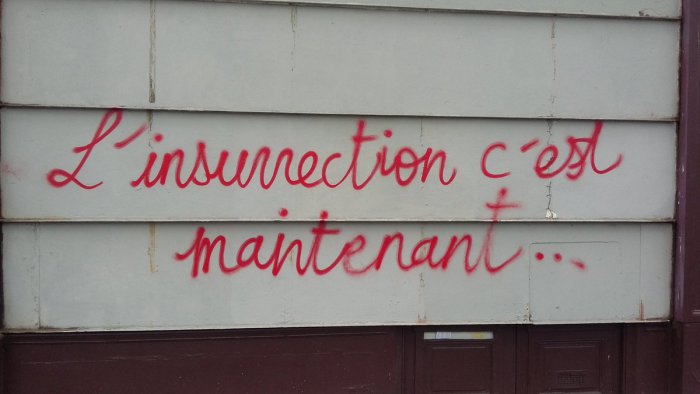This is a color photograph featuring graffiti on an outdoor wall. The upper part of the wall is composed of four panels of aged, white clabbered siding, displaying signs of corrosion. Below this section, the wall transitions into a brown area that appears metallic, tiling-like in parts, and extends to what could be mailboxes in the lower right corner, with one mailbox showing the edge of a paper sticking out. The white panels are spray-painted in red cursive text that reads "l'insurrection c'est maintenant..." which is French for "the insurrection is now..." The entire wall setup hints at an exterior possibly of a house or garage.